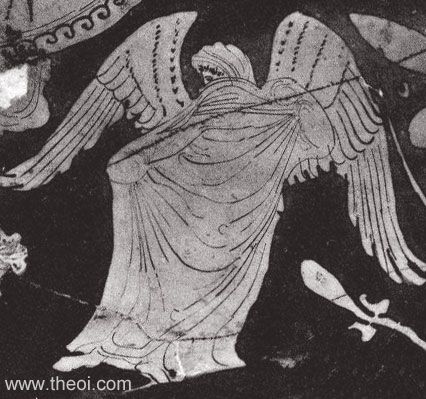The image is a black and white photograph, showcasing what appears to be an ancient piece of artwork, possibly Greek or Roman. Dominating the center of the composition is an angelic figure with large, outstretched wings. The angel is draped in a voluminous robe that covers most of its body, including the lower face and torso, giving the appearance of it being shrouded. The figure is positioned against a dark background, which highlights the lighter gray tones of the angel and the surrounding ornate and symbolic sections. Additional elements, like partial floral designs or other insignias, are visible but undefined. At the bottom left corner of the image, the text www.theoi.com is displayed, suggesting a connection to ancient mythology. The overall monochromatic scheme leaves it unclear whether the artwork itself is inherently black and white or if it was captured using a black and white camera.